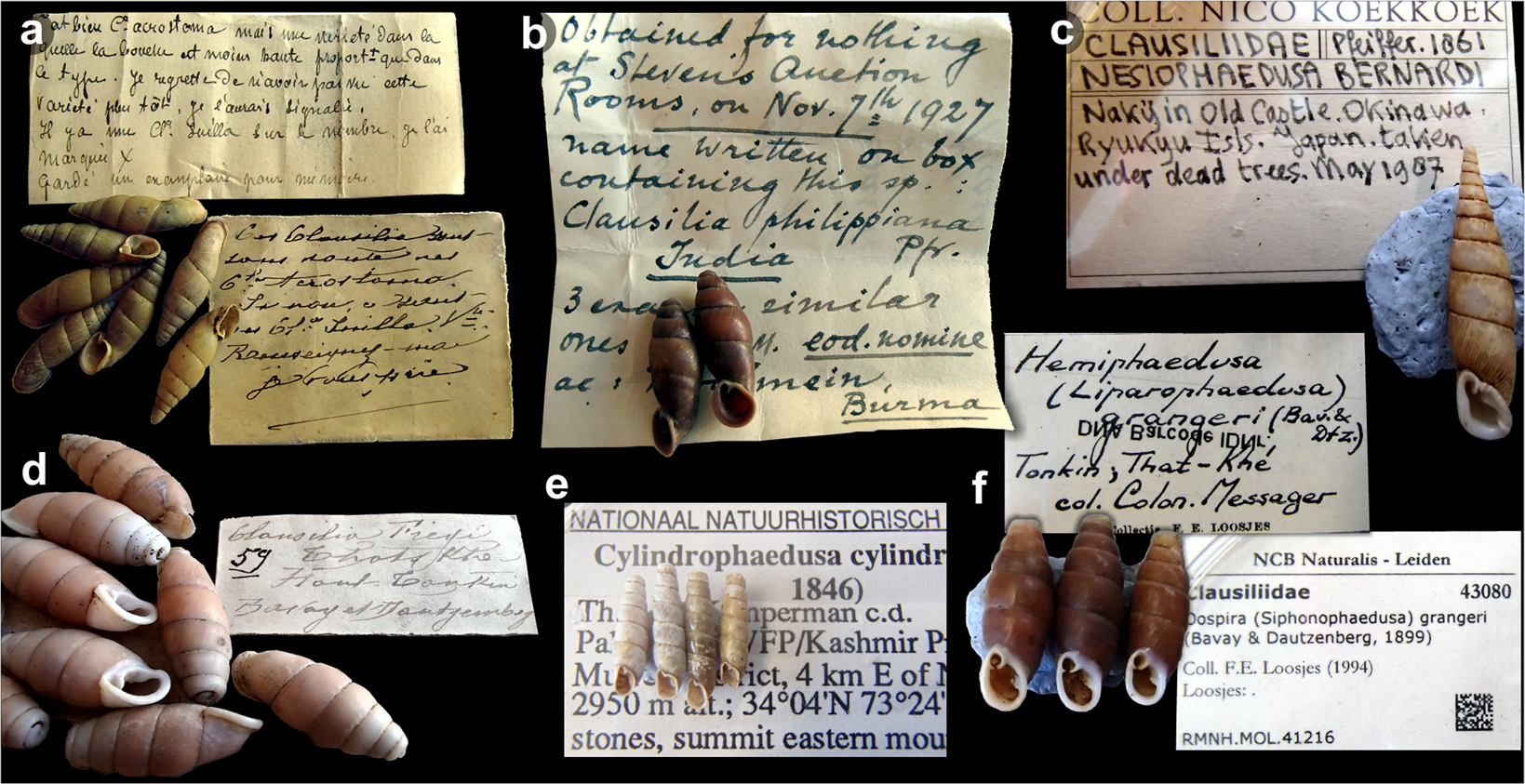This image depicts a meticulously curated display of seashells accompanied by descriptive notes on a black background, resembling a museum exhibit or content from a scientific textbook. There is a variety of seashells in shades of brown, pink, white, blue, and whitish-brown, some arranged in groups and others as single specimens. These shells are categorized and identified with handwritten and a few typed notes, noting details such as their type and the specific locations and dates they were found. There are a total of eight pieces of paper, some of which appear yellow, like sticky notes, while others are folded or formal cards. The notes are organized under labeled sections with letters A through F, detailing information such as "National Naturae Historica Cylindrical 1846 stone, summit of Eastern Mountain." This collection showcases a naturalist's meticulous record-keeping and the visual appeal of their seashell findings.